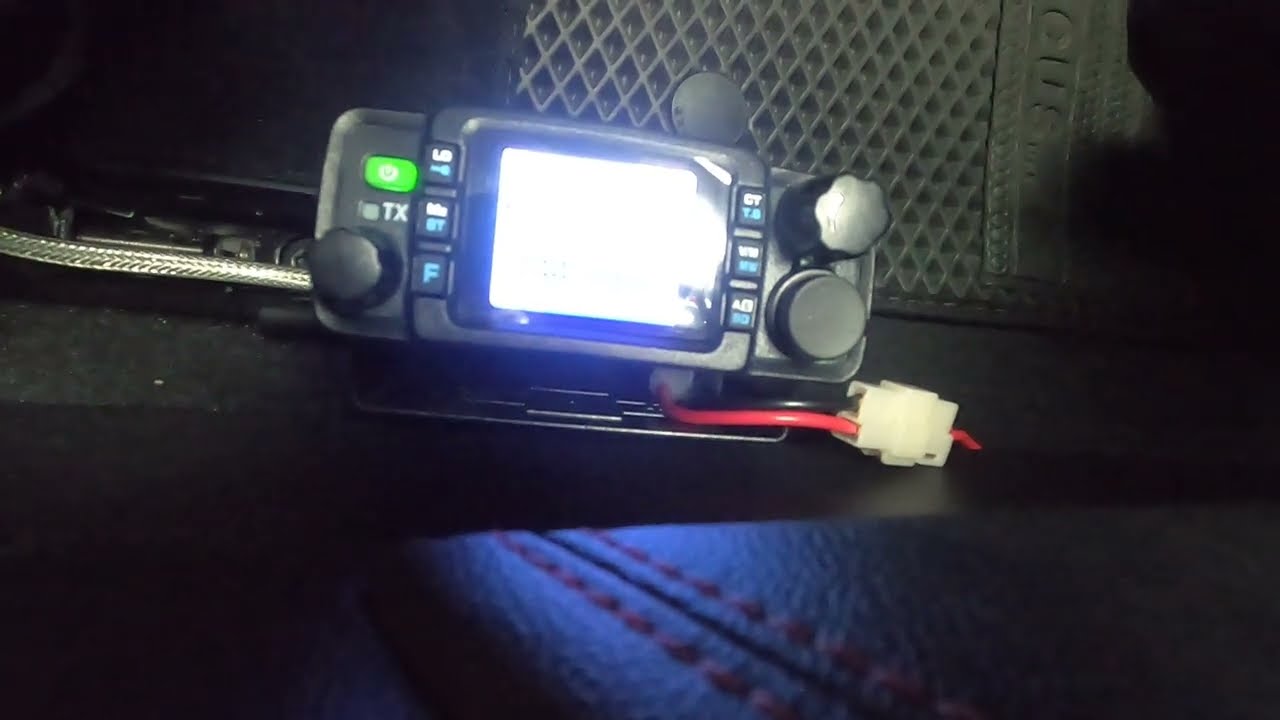The photograph depicts an electronic contraption, resembling a car stereo, lying on a dark, leather surface adorned with red stitching. The device is equipped with a prominent neon green power button, situated in the upper left corner, and a rectangular screen in the middle illuminated with a faint, blue-tinted white glow. The screen is flanked by three buttons each on its left and right sides, featuring white and blue text. Situated adjacent to the buttons on the right side are two black knobs, one of which is distinctively shaped like a flower. A red cable extends from the lower part of the stereo, headed towards the right. In the background, occupying the upper right portion of the image, is a black rubber mat with a diamond pattern and a vertical inscription. A silver cable emerges from the back of the device, trailing off to the left. The entire setup lies against what seems to be the floor or possibly the seat of a car, enhancing the impression of it being a car's interior.